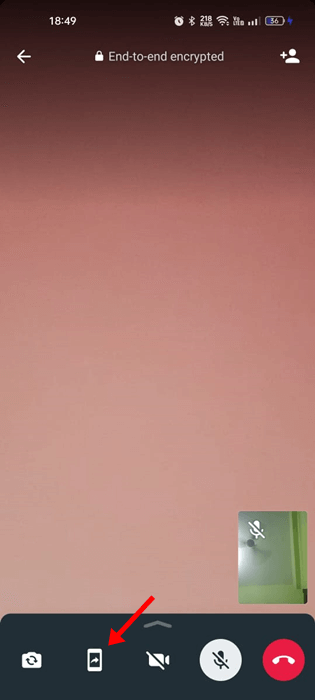The image shows the interface of a smartphone screen. At the very top left, an arrow icon points to the left, indicating a back function. Next to it on the right, the time is displayed as 18:49, followed by a series of status icons: an alarm clock, Bluetooth status, Wi-Fi signal with three or four bars, and a battery icon indicating approximately 34% charge remaining. Below these icons, there is a lock symbol and the text "end-to-end encrypted," suggesting a secure communication application. 

Beneath the status bar, a generic profile picture is shown with a plus sign next to it, possibly indicating an option to add a new contact or message participant. The background of the image transitions from a deep purple shade at the top, gradually becoming lighter towards the bottom. 

On the bottom right corner, a green-gray rectangle contains a microphone icon with a slash through it, indicating that the microphone is muted. On the bottom left, a white square with a white line in the middle is featured, and a red arrow points directly at this square from the upper right side, drawing attention to it.